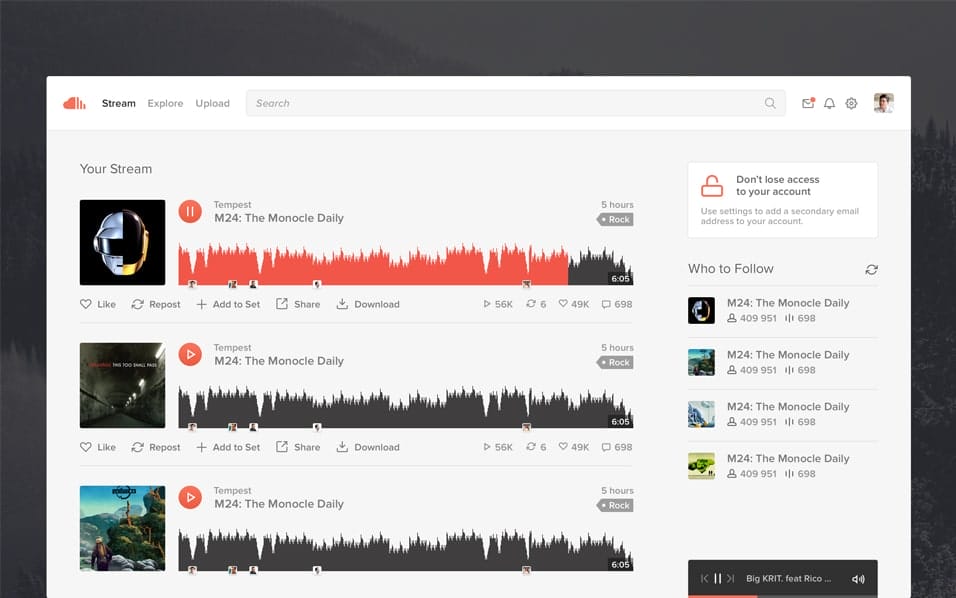This image displays a detailed view of a website called 'Stream' on a computer screen with a gray background. The main title "Your Stream" is prominently featured at the top. On the left side, there is a solid red icon, while the right side contains lines, adding to the design elements.

The central content includes information about "Tempest M24" in the 'Monocle Daily', accompanied by a fluctuating graph that resembles an EKG pattern, indicating fine, rapid movements in red and black bars. The graph spans across the middle of the screen, displaying time intervals up to five hours in gray on the right side. A notification banner suggests users add a secondary email for account security, indicated by a small lock icon.

Below the graph, there's a "Who to Follow" section, featuring three entries named 'M24' in the 'Monocle Daily'. Each entry has distinct images:

1. The first image shows a partially obscured face with half of it blacked out and the other half in blue with a touch of gold.
2. The second image is quite dark, possibly depicting a room with something shiny but details are indistinct.
3. The third image appears to be from a video game, showcasing a scene with rocks and a figure walking.

Each entry repeats the title 'M24 the Monocle Daily' and lists a time duration of five hours.